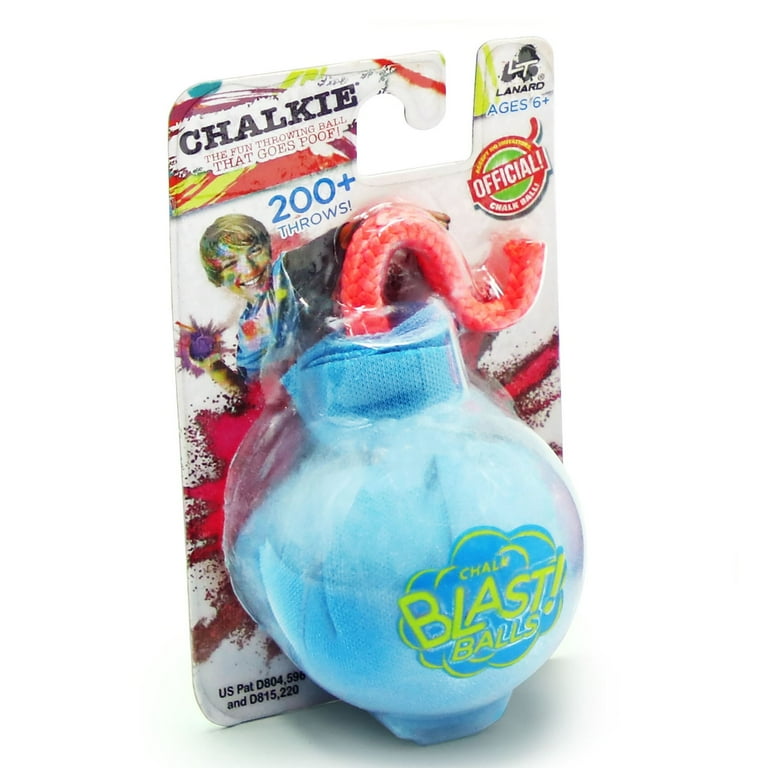The image depicts a children's toy named "Chalky," a fun throwing ball that goes "poof." The toy is encased in plastic bubble packaging affixed to a cardboard backing. The packaging prominently features the tagline "the fun throwing ball that goes poof," indicating the toy can be thrown over 200 times. A symbol on the packaging confirms it as an official Chalky ball, and the toy is recommended for ages six and up. The item itself is a light blue, roundish ball wrapped in a soft fabric, with a red string emerging from the top. The ball displays the text "Chalk Blast Balls" in neon green on a blue background. The packaging also includes an image of an excited child preparing to throw the ball. Additionally, the upper right corner of the package displays the brand name "Lanard" and a U.S. patent number is noted at the lower left.